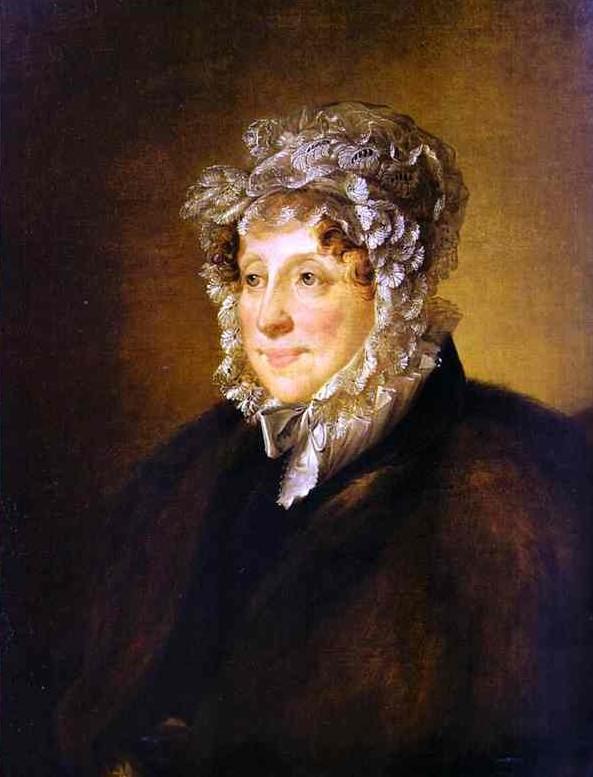This detailed portrait painting features a woman dressed in a remarkably elaborate white head covering that wraps from the top of her head down to a silver metallic tie beneath her chin. Her attire includes a baggy brown coat that exhibits broad white shoulders. The woman has a prominent, straight nose, heavy-lidded eyes that appear hazel or possibly blue, and slightly pink lips formed into a mild smile. Her red-tinted natural hair peeks out under the headpiece. She gazes off to the left with a bemused expression. The portrait captures her from slightly above the waist up, with a background that transitions from dark brown on the left to a lighter tan on the right, imitating the effect of candlelight.